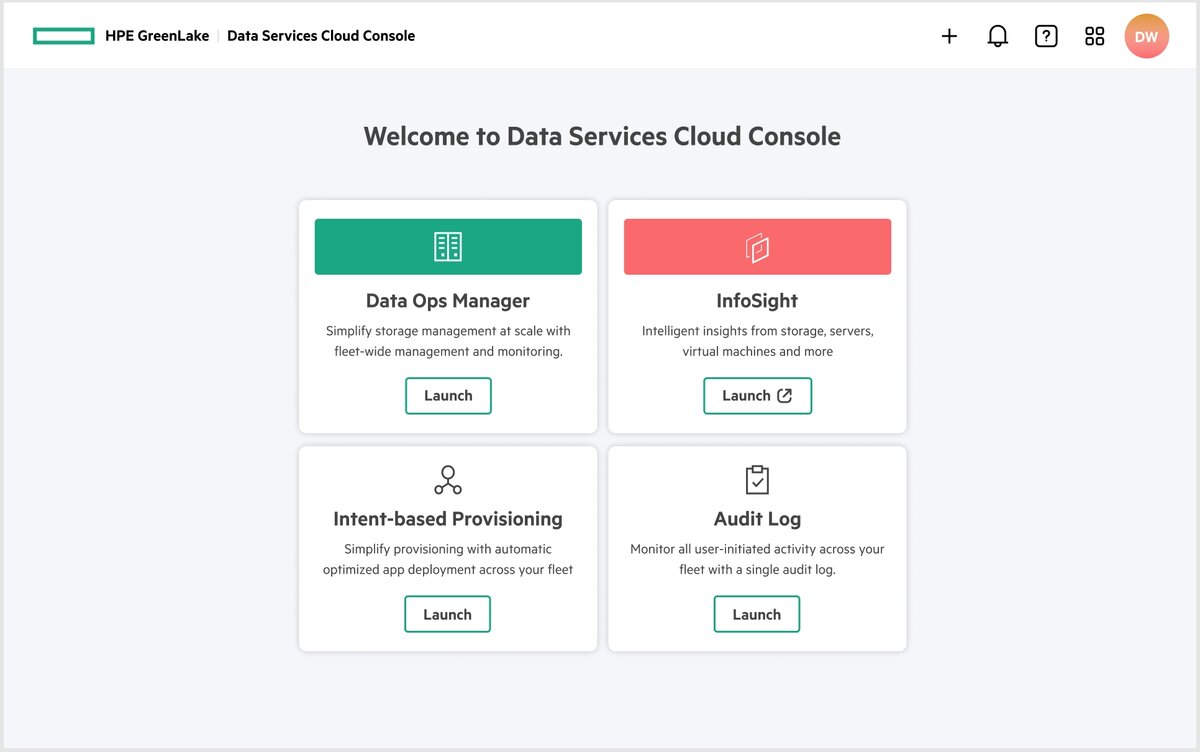**Descriptive Caption:**

This image is a screenshot from a website, encased in a thin black border. The top section of the image features a white strip approximately one inch in height, transitioning to a light gray background for the remainder of the image.

In the top white section, on the left-hand side, there's a long white rectangle outlined with a green border. To its right, in all capital black letters, is "HPE," followed by "GreenLake" in black text. A vertical line separates this from the next section. Adjacent to it, in bold black text, reads "Data Services Cloud Console." 

On the right side of this white strip, there's an orange circle containing the white letters "DW," with a four-square grid (two rows, two columns) inside. Additionally, there's the outline of a black square featuring a black question mark, followed by a notification icon resembling a black plus sign.

Moving to the center of the gray portion, bold black text announces, "Welcome to Data Services Cloud Console." Below this line, four modules are displayed in a 2x2 grid configuration.

- The top-left module features a green tab across the top and a small white square below it with horizontal lines, hinting at an icon. Bold black text labels this module "Data Ops Manager," followed by smaller text that reads, "Simplify Storage Management at Scale with Fleetwide Management and Monitoring." A white tab with a green border below this text contains the word "Launch" in black.
  
- The top-right module has a pink bar at the top, containing two overlapping squares. Below it, in bold text, is "InfoSight," accompanied by two lines of smaller black text. Like the previous module, it has a similar "Launch" tab at the bottom.
  
- The bottom-left module displays an icon of a circle with a branching line. The bolded title underneath is "Intent-Based Provision," followed by two lines of smaller text and a "Launch" tab similar to the others.
  
- The bottom-right module features a clipboard icon. Below it, in bold text, is "Audit Log," followed by two lines of smaller black text and the standard "Launch" tab at the bottom.

Each module is designed to stand out with its distinctive iconography, color-coded tabs, and clear, concise descriptions, likely indicating different functionalities or tools available within the Data Services Cloud Console.